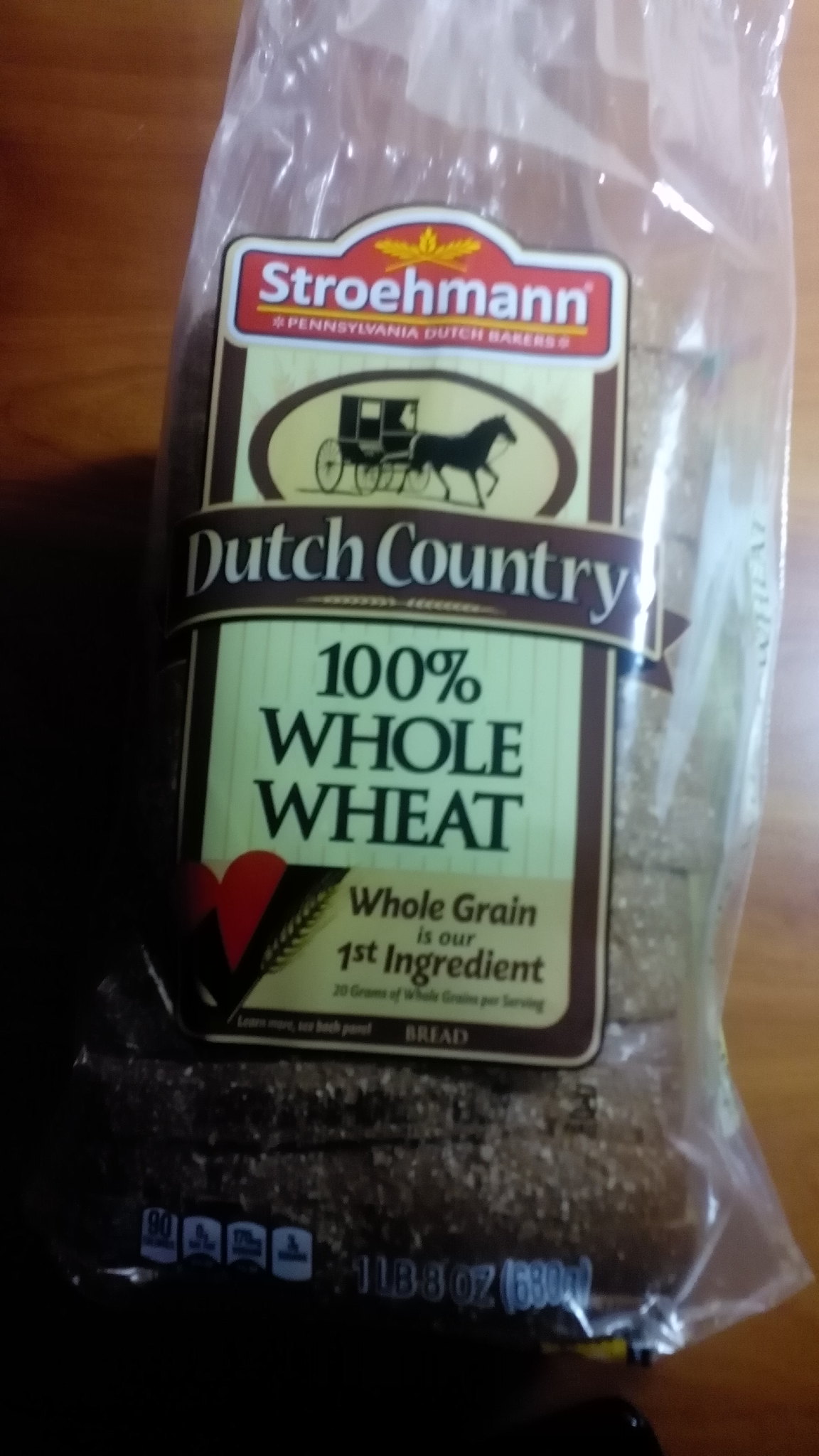The detailed image captures a close-up of a loaf of sliced whole wheat bread encased in a clear plastic bag, lying on a shiny brown wooden table. The packaging prominently features the brand name "Strohmann" in white letters on a red background at the top of the label, with three golden leaves forming an emblem above it. Below this is a yellow stripe, with the phrase "Pennsylvania Dutch Bakers" also in white. Centrally displayed is an off-white, cream-colored label bordered in brown, showcasing a dark brown oval containing a black illustration of a horse and buggy, reminiscent of Amish country imagery. Further down, "Dutch Country" is written in cream on a brown background, followed by "100% whole wheat" in bold black letters. In a light brown section towards the bottom, it states in brown lettering, "Whole grain is our first ingredient," with "20 grams of whole grain per serving" noted beside it. The bottom border contains nutritional details, including "90 calories" in blue among four small white circles. The clear bag allows visibility of the dark slices of bread, registering a weight of "one pound, eight ounces."